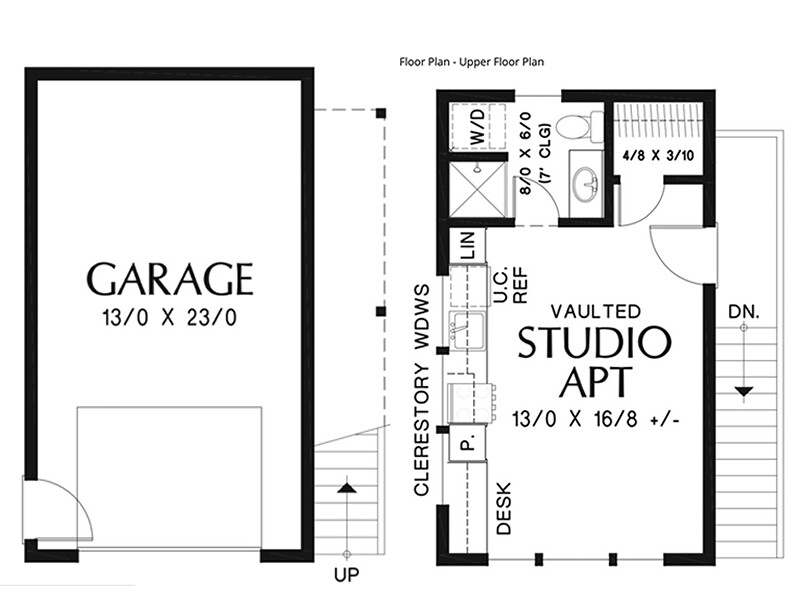The image depicts a detailed architectural drawing of a house design. On the left side of the drawing, there is a dark black outline. In the center, the word "Garage" is prominently displayed in black letters along with the dimensions "13'0" x 23'0". A lighter brownish square is positioned in the middle, near the entrance, indicating a specific area of interest.

Adjacent to this is what appears to be the main door, marked by a swish symbol on the left side. There are stairs indicated by an arrow pointing upwards. Also on the left, there is a dotted line accompanied by two square black dots.

Above the next section, "Floor Plan, Upper Floor Plan" is inscribed. To the side, some lettering reads "Cholesterol WDWS," although the exact meaning is unclear. Inside the layout, "Vaulted Studio Apartment 13'0" x 16'8" +/-" is written in black letters. A window seems to be represented near the desk area, which is marked with a line and two small black squares.

The upper floor features a black outline going upward with a door on the right and another door more centrally located to the left. The dimensions "4'8" x 3'10" are near this central door. Nearby, there is a bathroom represented with a sink, toilet, and the dimensions "8'0" x 6'0", accompanied by a note "7' CLG" indicating a 7-foot ceiling.

Within the bathroom, there is a washer/dryer (W/D) and possibly a bathtub. Adjacent to where the desk is located, there is an annotation "P." which likely stands for an appliance or possibly a sink or stove. "UC REF" indicates a refrigerator space, and a square box signifies the linen closet for the apartment.

Towards the exterior, a lighter gray outline depicts stairs with the label "DN" and an arrow pointing downwards, indicating a downward direction.